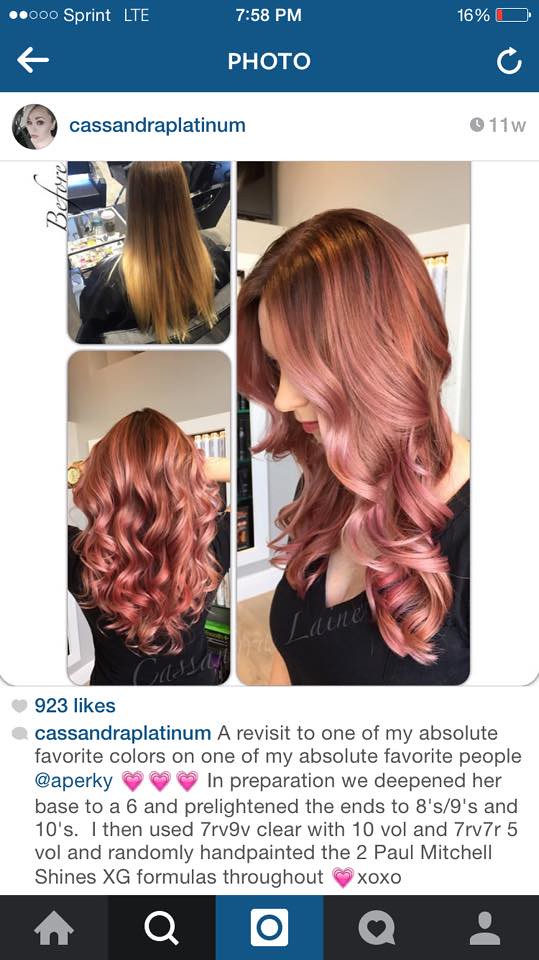The image is a color screenshot captured from a cell phone at 16% battery, showing an Instagram post by user Cassandra Platinum. At the top, a thick blue band displays mobile network details, connection type, time, and battery level. Below this, Cassandra Platinum's profile picture and username are located next to the word "photo" in white text centered on the blue bar. Three photos are displayed: two vertically stacked on the left and one larger vertical image on the right, all focusing on the intricate hairstyle of a woman with long, ornate red hair, styled to flow in curvy waves and facing sideways or away from the viewer.

The accompanying text, dense with hairdressing techniques, details how Cassandra revisited one of her favorite hair colors on a favored client at Aperkey. She explains deepening the base color to a level 6, pre-lightening the ends to levels 8, 9, and 10, and using a mix of 7RV9V clear with 10 volume, and 7RV7R5 volume. The process involved randomly hand-painting using two Paul Mitchell Shrine XG formats, emphasizing the meticulous and personalized approach to the hair work. The post has garnered 923 likes, as indicated by the heart symbol and like count below the images, followed by a comment section suggesting interaction by the same poster. The bottom of the screen shows various navigation icons in black, suggesting it is within a standard Instagram user interface.